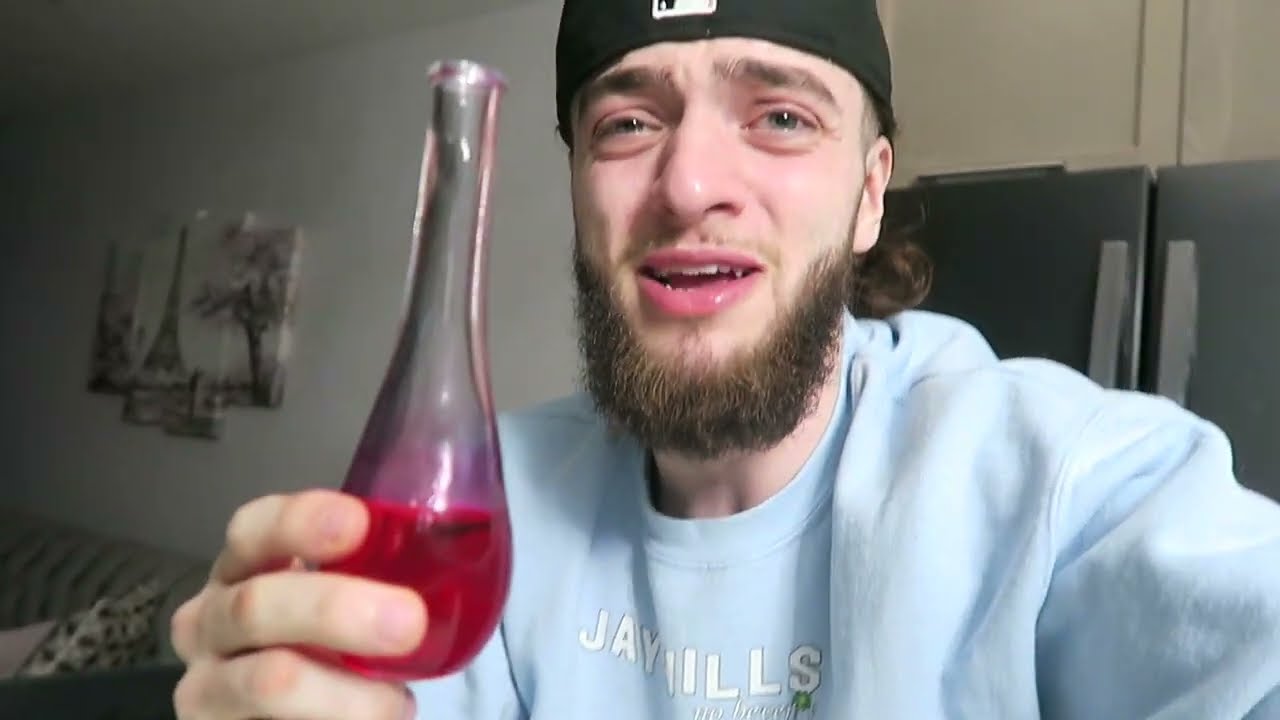A young man, possibly in his twenties, stands facing the camera, appearing to speak with his mouth open. He wears a backwards black baseball cap with a small black and white logo on it and has a scruffy brown beard along his jawline and a stubbly mustache. His eyes appear gray. The man is dressed in a light blue long-sleeve sweatshirt with the partially visible white text "JAVI LLS" or "J. Hills" printed on the front. In his right hand, he is holding a glass container with a rounded base filled with red liquid, resembling a test tube or a chemistry set vial. The background features a bare white wall with a double-sided gray or silver refrigerator. On the left side of the image, a portrait of the Eiffel Tower hangs on the wall above a striped couch with a pillow.